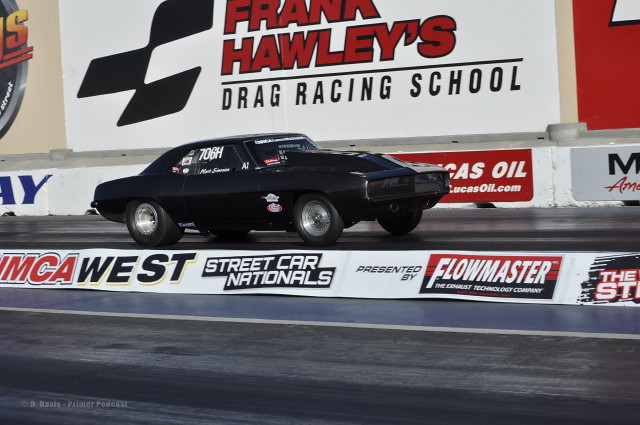This vibrant color photograph captures a sleek black race car poised at a racetrack, ready for the Street Car Nationals event. The foreground prominently features the black car adorned with sticker decals, including a distinct "706H" on the passenger side window amid smaller, unreadable text. Surrounding the car, multiple advertisements are strategically positioned, enhancing the dynamic atmosphere of the scene. Directly below the car, a white low wall bears the bold, red and black text, "YMCA West Street Car Nationals, presented by Flowmaster," alongside a logo. In the background, a second white wall filled with more advertising can be seen, though specific details are obscured. Notably, "lucasoil.com" stands out, indicating sponsorship. Centered above the scene, a large advertising sign in red text reads, "Frank Hawley's Drag Racing School," contextualizing the setting within the high-energy environment of a drag race about to commence. The vivid colors of white, black, and red in the advertisements underline the event's vibrancy and sense of anticipation.